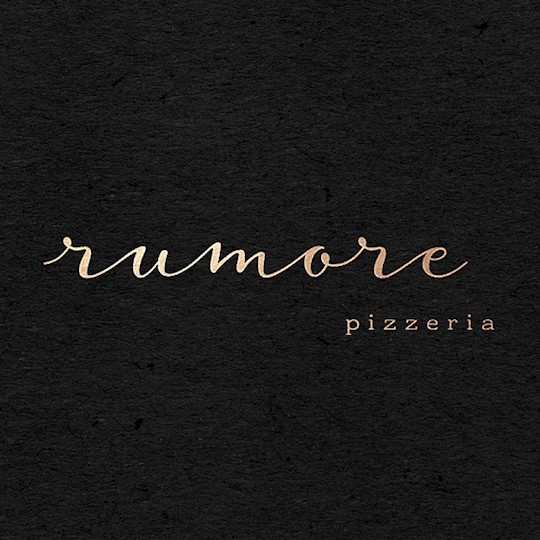The image showcases a central text-based logo for "Rumor Pizzeria" against a textured black background with subtle gray highlights, resembling grainy wood or paper. The word "Rumor" is prominently written in an elegant cursive style with flowing, connected letters, placing emphasis on a sophisticated yet inviting brand presence. Just below "Rumor," positioned slightly to the right, the word "Pizzeria" appears in a contrasting, simpler typeface such as Times New Roman, providing a clear and readable descriptor for the restaurant. The colors used are primarily a light gold or goldish-brown for the text, which stands out against the textured dark background, giving it a distinguished and classy look, ideal for a business card or signage.